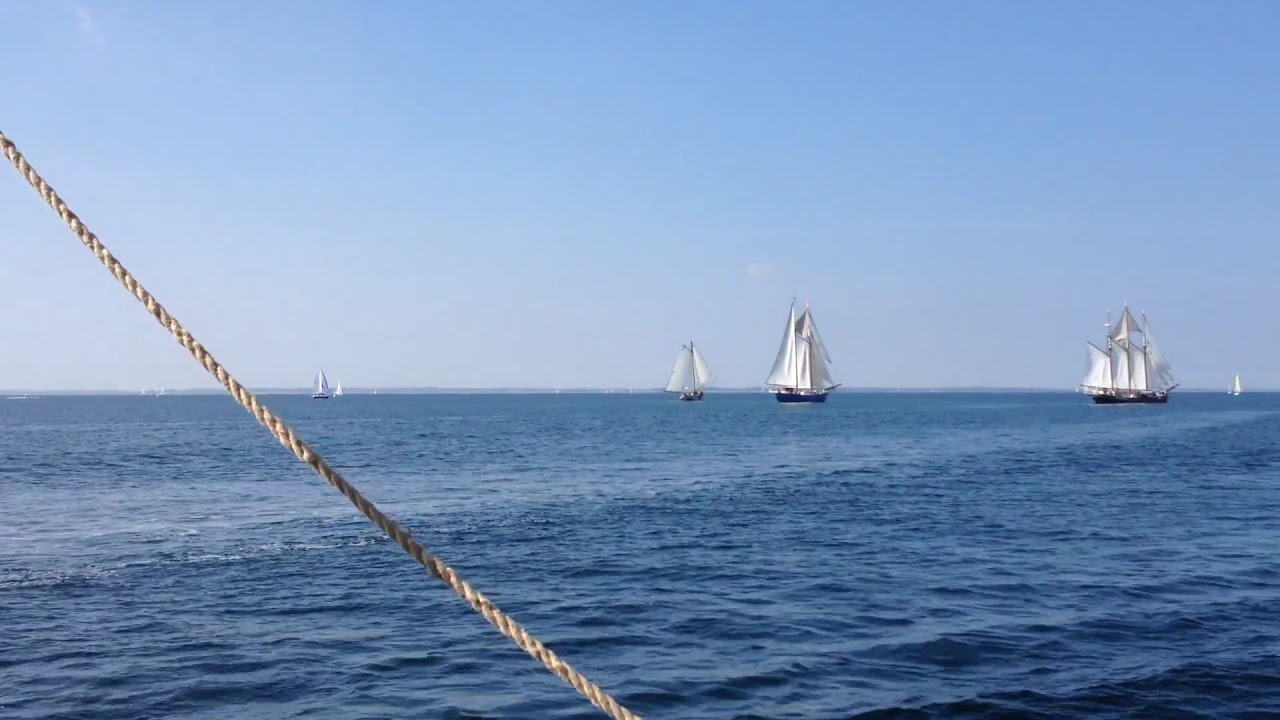A captivating photograph captures a serene ocean scene under a light blue sky tinged with whitish-gray along the horizon. Dominating the expansive blue waters are several tall ships with white sails gracefully cutting through the slightly choppy, yet relatively calm waves. In the foreground, a ship's rope descends diagonally from the top left to the bottom center of the image, framing the maritime tableau. 

The composition features three prominent sailing vessels: the largest ship with four majestic masts and numerous sails occupies the right-hand side, while a medium-sized ship with three sails drifts towards the center. Nestled between these is a smaller ship centrally positioned, with additional distant ships faintly visible against the horizon, appearing as tiny triangles. Notably, a lighthouse-like tower stands to the right of the large ship, adding a quaint coastal touch to the scene. Though the photo's perspective remains ambiguous, the sun's angle suggests it's shot in mid to late afternoon, casting a gentle light over this tranquil oceanic vista.